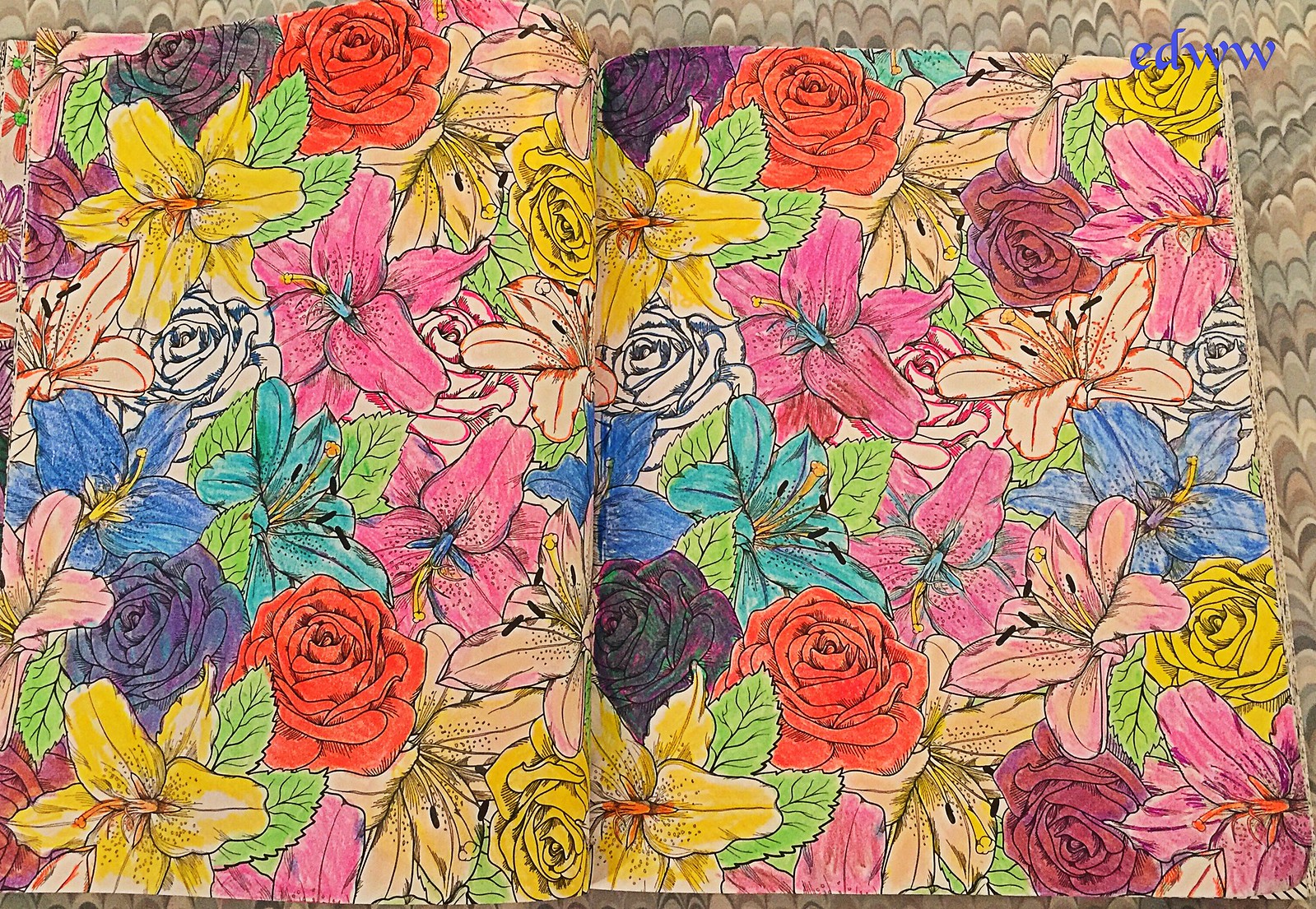The image is a detailed, color photograph featuring what appears to be a page from a coloring book that has been partially colored in. The design showcases a variety of flowers, including roses, tulips, and lilies, with most of them fully colored. The colors used are predominantly pinks, reds, yellows, and greens for the leaves. However, some parts of the page are still left clear or only lightly outlined. In the right corner of the image, the initials "EDWW" are visible, written in a cursive purple font. The overall presentation of the page, combined with the flatness and slight fold indications, suggests that this could also be a decorative piece such as gift wrap or scrapbook paper, possibly intended for sale on a website, indicated by the "EDWW" branding. The backdrop behind the floral design consists of a simpler, modern brown pattern.